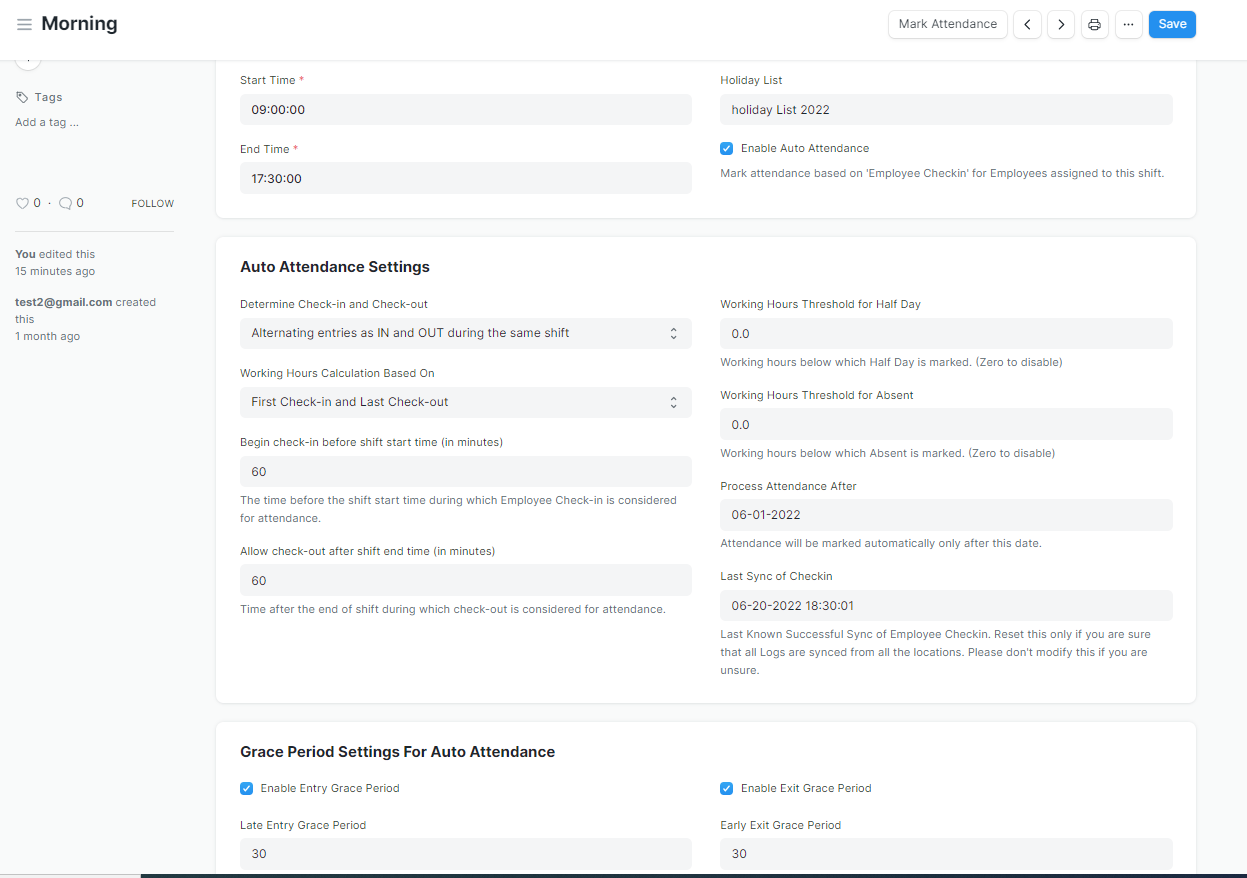Screenshot of Attendance Information Page

This screenshot captures a detailed view of an attendance information page. At the top, the word "Morning" is prominently displayed in black text against a white background, accompanied by three horizontal lines that presumably function as a clickable menu.

To the right of this section, several buttons are arranged neatly: "Mark Attendance," left and right navigation arrows, a three-dot button likely used for settings, and a "Save" button.

Beneath this, on the left side, there are tags featuring a heart symbol and a speech bubble icon, both showing a count of zero. Additionally, there's an option to follow the page.

To the right, detailed information is present, starting with "Start Time" listed as 09:00 and "End Time" as 17:30. Below this, there's a "Holiday List" section indicating "Holiday List 2022" with an option to enable auto attendance. Following this, there's an "Auto Attendance Settings" area containing multiple text boxes for user input.

Towards the bottom of the page, "Grace Period Settings for Auto Attendance" offers further configuration options related to attendance management.